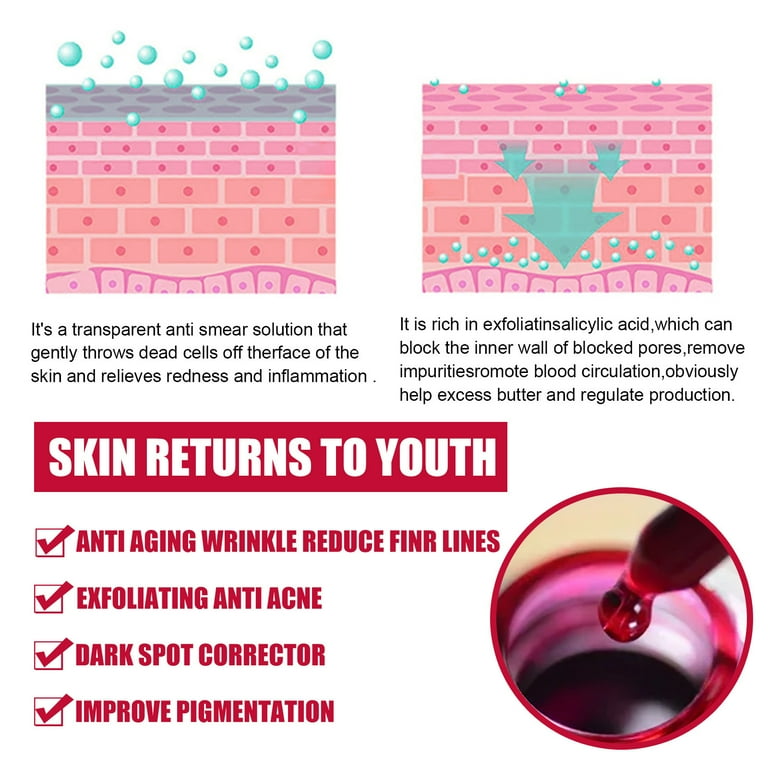This advertisement showcases a powerful skincare product designed to rejuvenate the skin. The top section of the ad features two illustrative diagrams against a white background. On the left, a graphic displays the skin's layers with large blue bubbles emerging from the surface, symbolizing the product's transparent anti-smear solution. This solution gently exfoliates by removing dead skin cells and alleviating redness and inflammation. The right graphic shows small droplets being absorbed deeper into the skin layers, highlighting the product's rich salicylic acid content. This ingredient effectively unblocks pores, removes impurities, boosts blood circulation, helps manage sebum production, and promotes balanced skin.

Beneath these diagrams, a prominent red rectangle with bold white text announces that "skin returns to youth." This section lists key benefits with checkmarks for easy reference: anti-aging wrinkle reduction, finer lines reduction, exfoliation with anti-acne properties, dark spot correction, and improved pigmentation. To the right, a circular inset visualizes the product's application, depicting an eyedropper releasing a drop of red liquid into a red bottle cap.